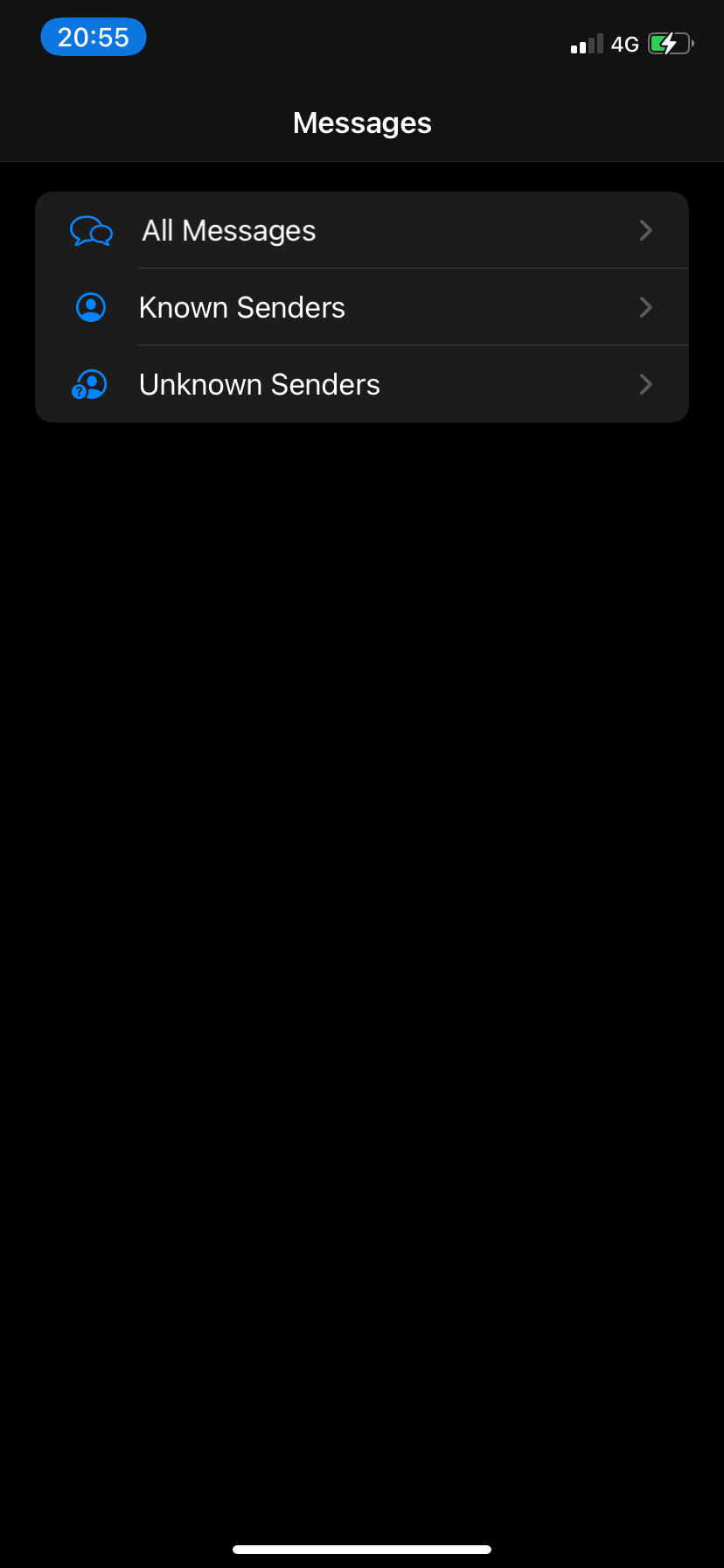This image displays a screenshot of a messaging app's settings page, configured in dark mode. The interface prominently features a deep black background, paired with a gray top border and text areas, creating a visually distinct and modern look. 

In the lower half of the screen, a thin white line stretches horizontally, likely indicating the area where users can swipe up to close the app. At the top of the screen, the status bar is visible: on the left side, a small blue bubble displays the time as 20:55 in white text; on the right, a signal indicator shows two out of four bars with "4G" next to it, and a battery icon is half-filled in green with a white lightning bolt, signifying that the device is currently charging.

Directly below the status bar, bold white text reads "Messages," followed by three sub-options: "All Messages," "Known Senders," and "Unknown Senders." Each of these options is accompanied by a right-facing gray arrow, suggesting they are clickable for more detailed settings. Accompanying icons to the left of these options enhance clarity: a pair of speech bubbles for "All Messages," a profile silhouette for "Known Senders," and a profile silhouette with a question mark for "Unknown Senders." The clean design and intuitive icons make navigation straightforward and user-friendly. 

Overall, this caption provides a thorough and vivid description of the messaging app's settings page in dark mode.